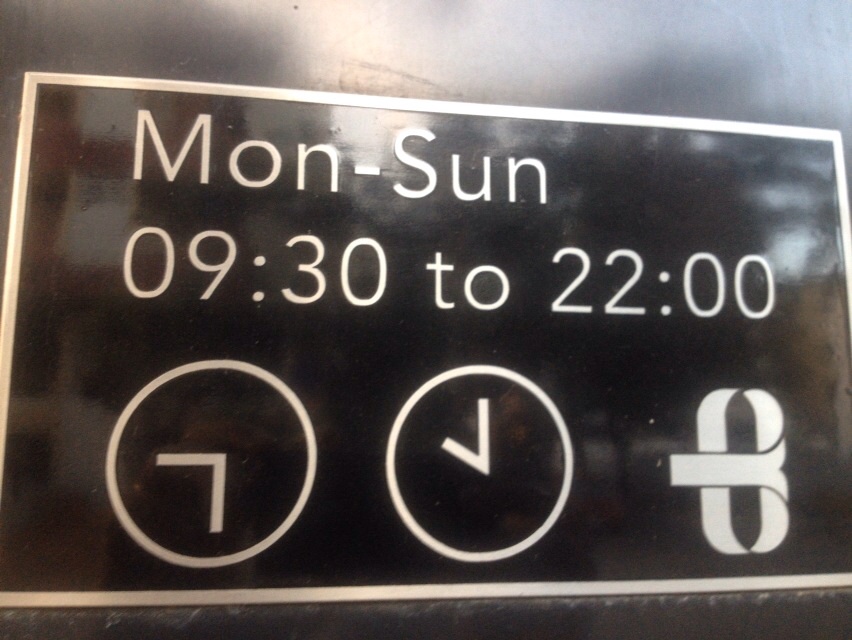The image is a reflective black sign bordered in white. In the center, white text indicates operation hours: "Mon-Sun 09:30 to 22:00," suggesting a non-U.S. location due to the 24-hour format. Flanking the text are two minimalist clock icons, one displaying 09:30 and the other 22:00. To the right, a symmetrical white logo resembling an 'O' with a central slash and ribbon-like extensions is visible. The reflective surface hints at glass or marble, capturing indistinct reflections of surrounding lights.